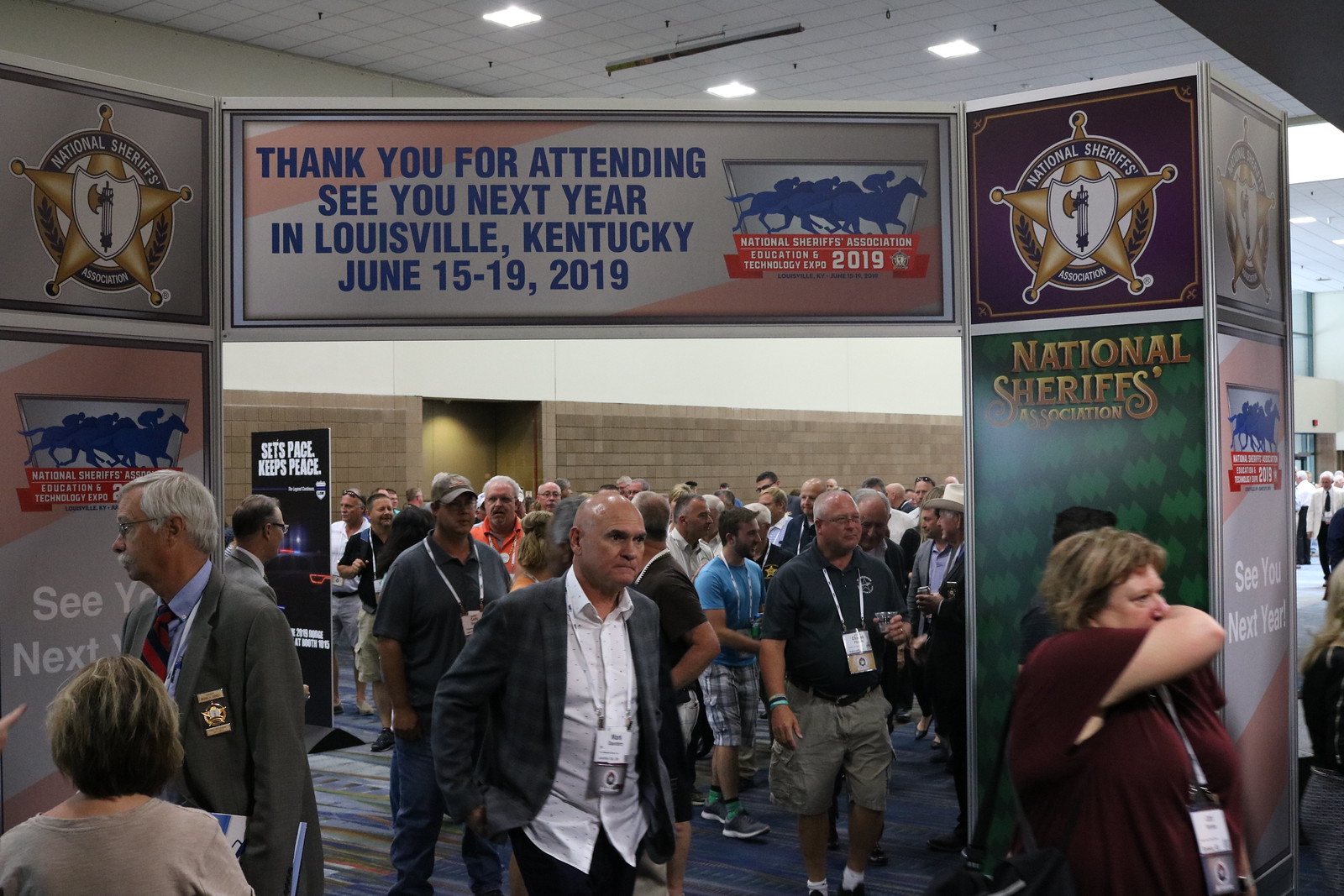The image captures a bustling scene at the National Sheriffs Association Education and Technology Expo 2019. Attendees, many with lanyards and identification tags around their necks, fill the predominantly blue and gray carpeted room. At the center, a man in a gray suit with an open white-collared shirt stands out among the crowd, as does another man in cargo shorts and a dark polo shirt. The room seems to be part of a larger conference or office building, illuminated by white spotlights overhead. Prominently displayed are two large square signboards connected by a center banner. The left signboard features a logo of riders on horses above a red banner. A small silver square with a star logo indicating the National Sheriffs Association sits above it. The central banner reads, "Thank you for attending. See you next year in Louisville, Kentucky, June 15-19, 2019," and is flanked by repeat logos of riders on horses. The right signboard mirrors the left, topped with a purple square and the recurring symbol. The sense of community and anticipation for next year’s event in Louisville is palpable in this well-attended gathering.